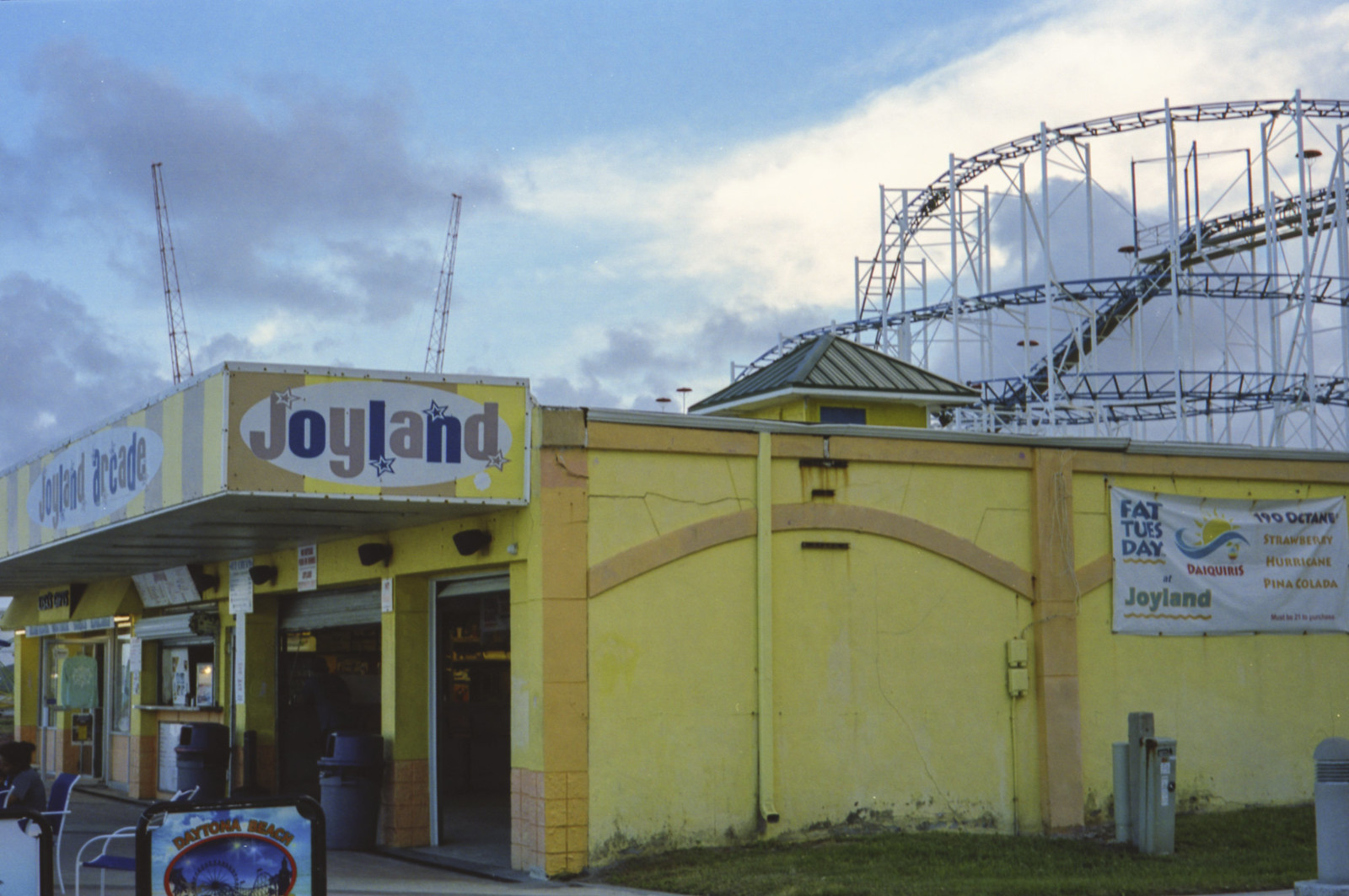The image depicts an older, vibrant yellow and orange building labeled "Joyland," featuring an awning with "Joyland Arcade" prominently displayed on the front. The facade includes open bay windows, a service window, and several doors, creating a busy frontage. In front of the building, there are two trash cans, and a sign for "Daytona Beach." On the middle right side, another sign reads "Fat Tuesday at Joyland" with details about daiquiri flavors like 190 Octane, Strawberry Hurricane, and Pina Colada, beside an illustration of a yellow sun and a blue wave. To the right, past a grassy area with some chairs—blue and white ones, with one person seated—a white roller coaster track is visible against a sky transitioning from light blue to dark blue, scattered with gray and white clouds. The setting appears to be at dusk, adding to the nostalgic and slightly weathered charm of the scene.